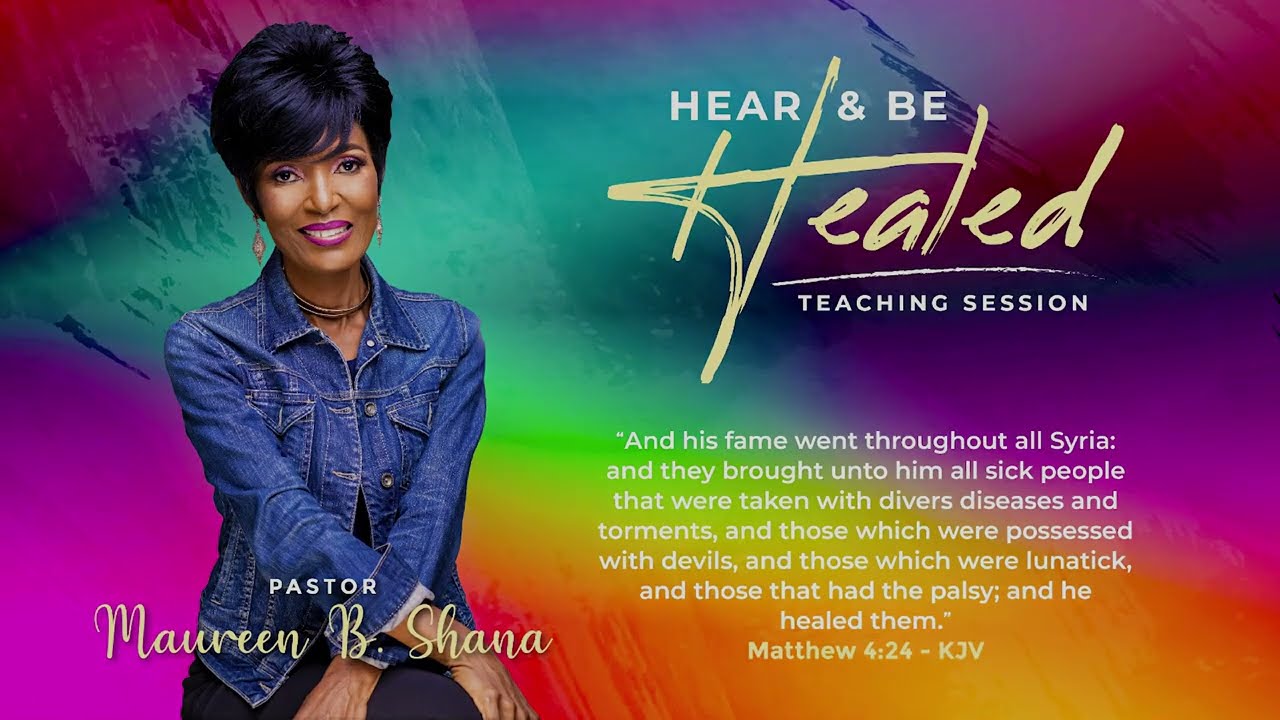The poster advertises a teaching session titled "Hear and Be Healed," featuring Pastor Maureen B. Shana. The design is vibrant, with a colorful background featuring swirling shades of purple, orange, pink, blue, green, yellow, and red. The event's central theme focuses on healing, supported by a Bible verse from Matthew 4:24 (KJV) that states, "And his fame went throughout all Syria: and they brought unto him all sick people that were taken with divers diseases and torments, and those which were possessed with devils, and those which were lunatic, and those that had the palsy; and he healed them."

The image of Pastor Maureen B. Shana is prominently displayed. She is a glamorous African American woman with ear-length black hair, wearing bright pink lipstick. She is dressed in a denim jacket, accessorized with a large necklace and big, diamond-shaped earrings. Her pose is confident and engaging, with her hands crossed over her knee and a knowing glance directed at the camera. The text "Hear and Be Healed" is creatively styled, with "Healed" in a distinct cursive yellow font, while the rest of the text, including "Teaching Session," is in white.